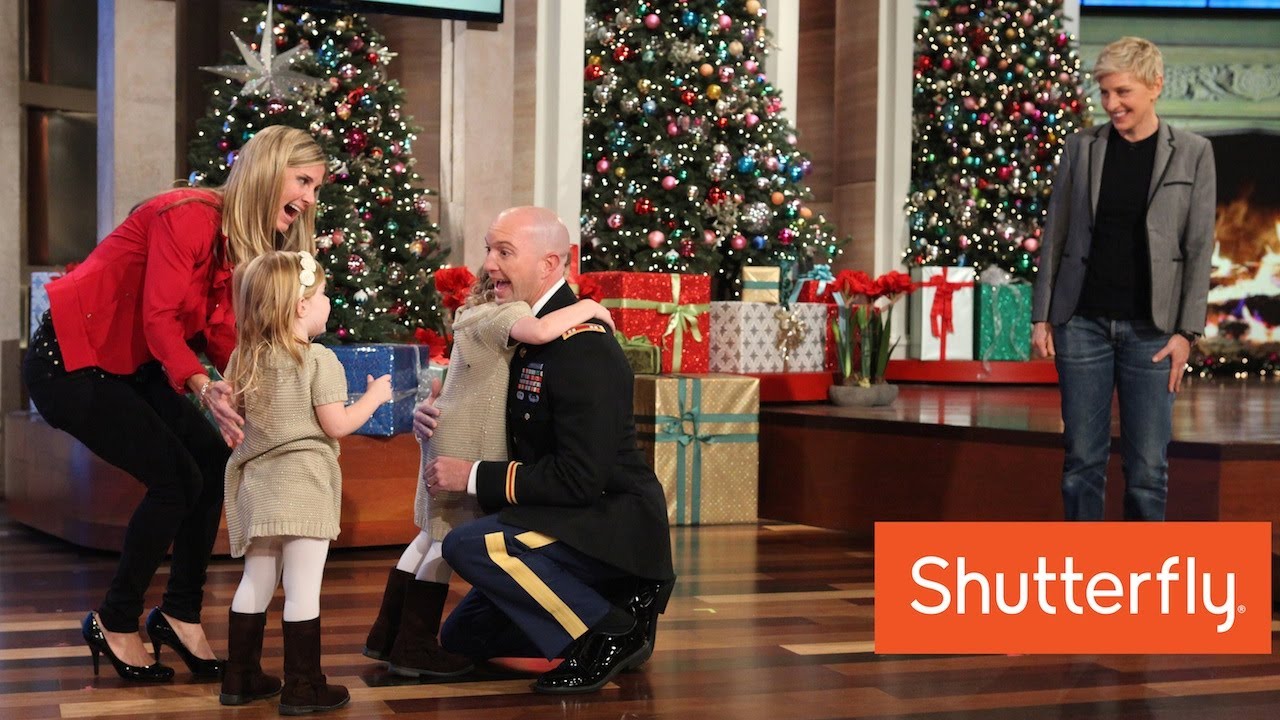In this high-quality image from the Ellen DeGeneres Show, copyrighted by Shutterfly, a heartwarming family reunion unfolds against a festive Christmas backdrop. On the far right, Ellen DeGeneres watches with a smile, dressed in blue jeans, a black T-shirt, and a grey work jacket. The set features a roaring fire encased in a lime-green fireplace, three lavishly decorated Christmas trees adorned with assorted ornaments, and an array of wrapped presents scattered beneath them and in the background. The floor is a multicolored wooden design that adds warmth to the scene.  

To the left, a woman with blonde hair, dressed in a bright red jacket, black trousers, and high-heeled shoes, beams with joy as she stands near her two young daughters. The girls, who appear to be twins, are wearing matching beige sweater dresses with white leggings and black boots. A bald man, likely a service member of the Royal Navy, is central to the scene, donning a distinguished uniform complete with various badges, a black overcoat, blue trousers with a yellow stripe, and shiny black shoes. He embraces one of the daughters while the other eagerly awaits her turn. An orange rectangle at the bottom right corner of the image features the Shutterfly logo, marking their sponsorship of the touching moment.